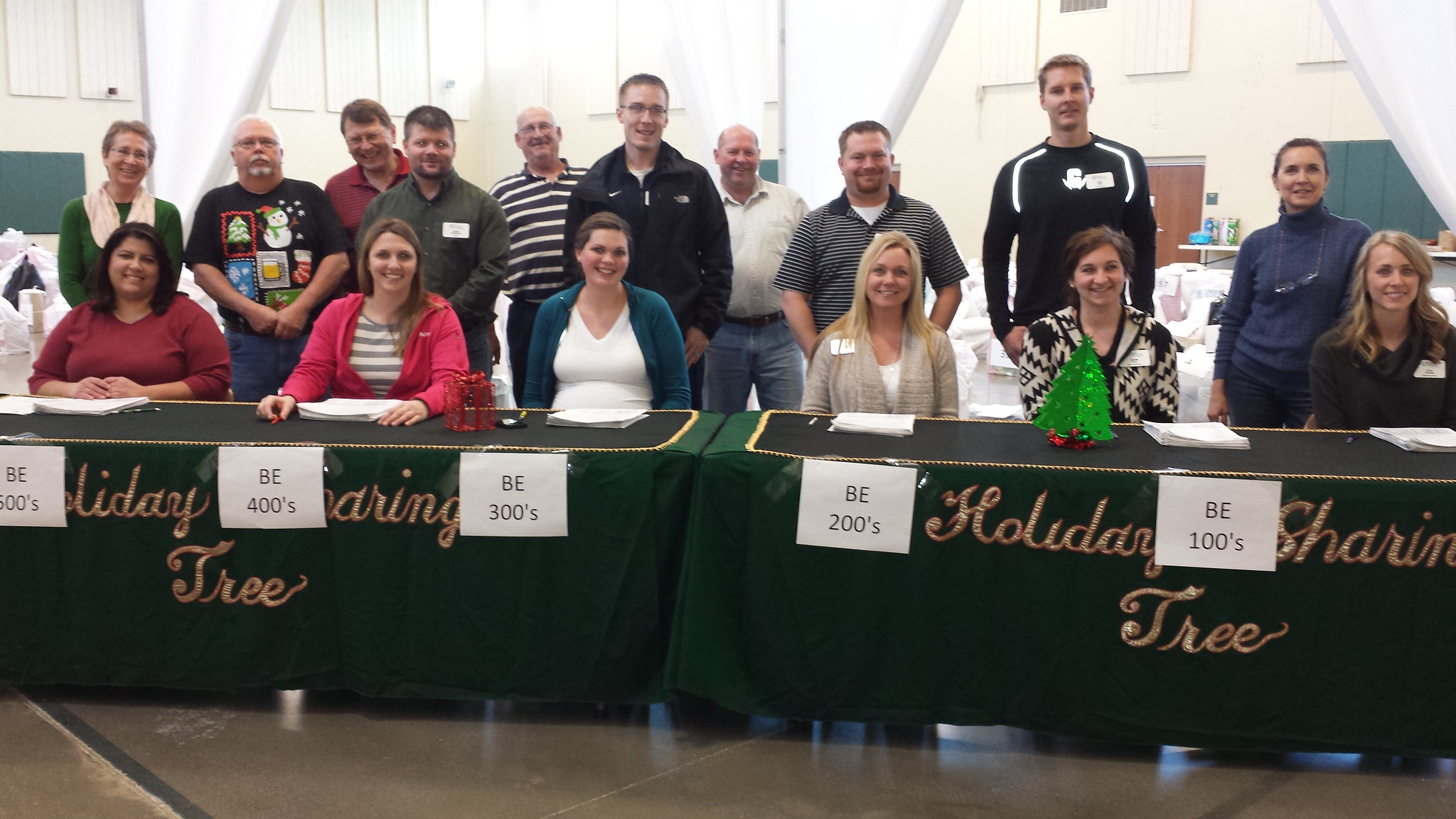The image is a color photograph of an event featuring two tables, each covered with green tablecloths and adorned with gold cursive text reading "Holiday Sharing Tree." The tabletop has a black mat bordered in gold. Affixed to the front of the tables are five evenly spaced printouts labeled "BE 100s," "BE 200s," "BE 300s," "BE 400s," and "BE 500s." Seated behind these tables is a row of women, each with papers in front of them. Beside a small Christmas tree on the right table, a group of mixed-gender individuals stands behind the seated women. The setting appears to be a large indoor space, possibly a gymnasium, with beige walls and visible wall padding, indicating a school event or community gathering.